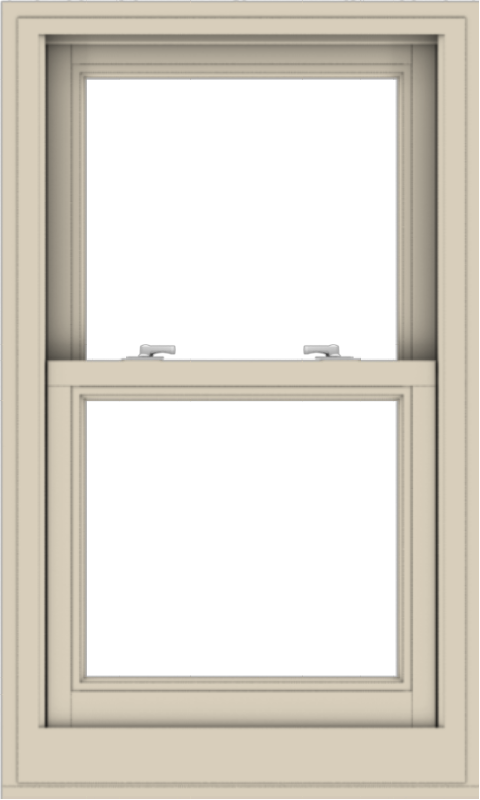This image depicts a rectangular window with a beige, wide-framed pull-up design, featuring two panes, one above the other. The window's height is longer than its width. There are two silver locks, or handles, on the top of the bottom pane, which are facing each other and ensure that the window remains closed and locked. The exterior frame appears slightly lighter than the interior frame, which is more of a tan beige color. The window's background is bright and white, making it impossible to see through the glass. There is a ledge at the bottom of the window, and the overall aesthetic is one of simplicity and functionality, with the panes presenting a clean, white appearance.